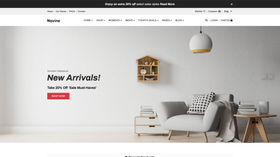A very small, blurry screenshot featuring several indistinct elements except for the central left text that says "NEW ARRIVALS!" in black. The top of the page has a black bar with illegible writing, followed by a white navigation bar with multiple categories on either side. Below this is another bar featuring an indistinct dark black word, alongside seven tabs in the middle and three on the right, all unreadable. 

The main portion of the screen displays a modern, minimalist interior of a home or apartment with white walls and flooring, bathed in natural light. The focal point is a white, puffy chair with a black and white patterned pillow. Adjacent to the chair is a small, round modern light-tan wooden table adorned with white objects, possibly books or decorative items. To the left stands a matching bedside table with a white front and two drawers, holding additional white decorative objects. Above these furnishings is a small, house-shaped shelf with five compartments holding various unidentified knick-knacks. Adding to the modern aesthetic, a white, round pendant light resembling a glowing orb hangs above the chair, featuring a subtle yellow tint at its bottom edge.